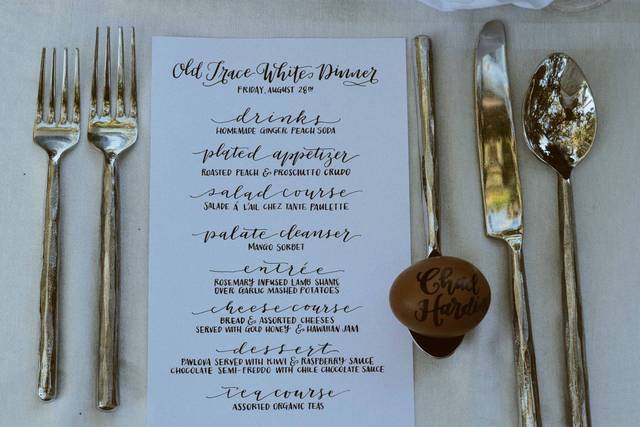The image depicts an elegant place setting for a formal dinner event on a white tablecloth. Positioned centrally on the table is a white paper menu with details of the meal, categorized in cursive for the courses and in a more readable font for the food items. On the left side of the setting are two forks: a slightly smaller salad fork and a larger dinner fork. On the right side, there is a butter knife, a large spoon, and a small spoon inverted with a red hard-boiled egg resting on it, which has cursive writing, likely a name, inscribed. The menu announces "Old Trace White's Dinner, Friday, August 28th" and lists the courses to be served: homemade ginger peach soda for drinks, a roasted peach and prosciutto crudo plated appetizer, a salad course of salad à la Che, a mango sorbet palette cleanser, an entrée of rosemary-infused lamb shank over garlic mashed potatoes, a cheese course with bread and assorted cheeses served with gold honey and Hawaiian jam, and desserts featuring pavlova served with kiwi and raspberry sauce, along with chocolate semifreddo with chili chocolate sauce. The meal concludes with a selection of assorted organic teas.